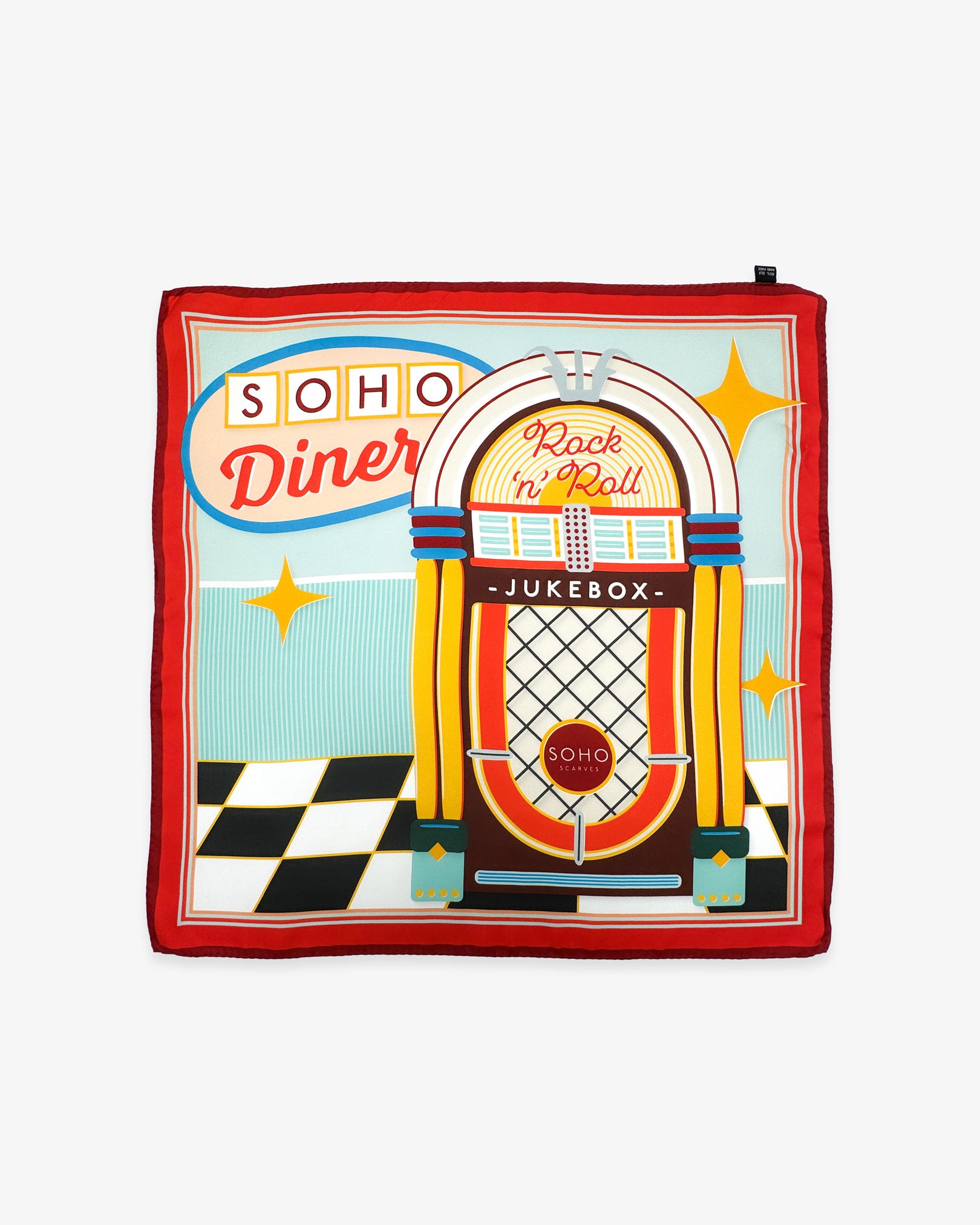This image portrays a retro-themed, square-shaped cloth with a vivid red border and a finer internal border comprising a thin red and orange line. At the center of the cloth, there's a highly detailed illustration reminiscent of a 1950s diner advertisement or napkin. 

The focal point is an old-fashioned jukebox with a distinctively curved top. The jukebox has a prominent, white arch adorned with a W-like gray design, flanked by yellow and red stripes on either side, and features songs selection dials in a contrasting mix of blue with yellow separators. A black background across the midsection bears the word "Rock and Roll" in white letters, and directly beneath, "Jukebox" in a similar style. The jukebox sits on a classic black and white checkerboard floor, bordered by yellow.

The backdrop of the jukebox scene is divided horizontally at the midsection: the lower half is a darker blue while the upper half is a lighter blue. Towards the upper-left corner, the setting is marked by an oval pink sign, outlined in blue, that states "Soho Diner". Inside the oval, the word "Soho" appears in separate white-backgrounded boxes, with each letter in burgundy red, while "Diner" is displayed below in a distinct red script.

Three yellow star-shaped designs sporadically decorate the gray background of the cloth, enhancing the vintage aesthetic. Additional decorative elements include three yellow diamonds on the wall and blue lines with interspersed red accents flanking the jukebox, with the lower part exhibiting a gradient of dark to light green. Overall, this design is a vibrant homage to mid-century American diner culture.